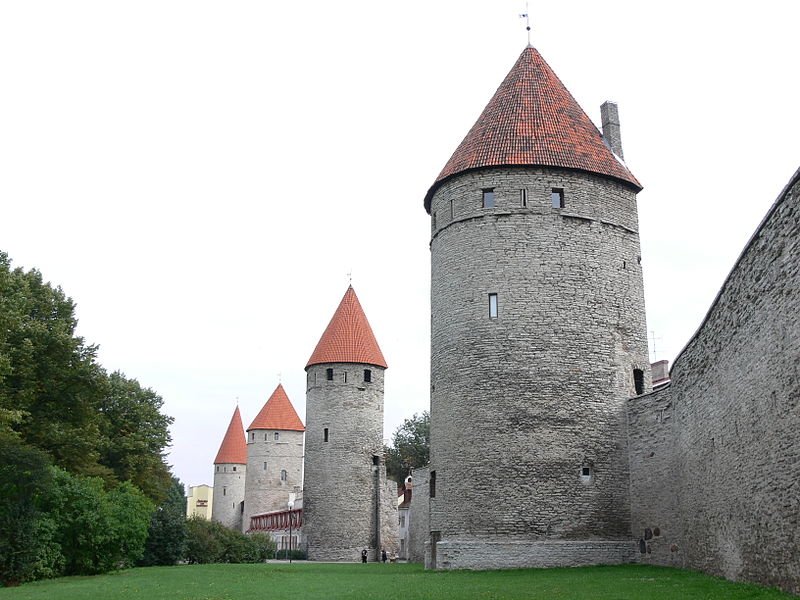This vertical rectangular image captures an outdoor scene dominated by a castle-like stone wall, featuring four turrets. These cylindrical turrets, constructed from a blend of light and dark gray older stone, vary slightly in size but are uniformly topped with metal cone-shaped roofs in a mix of black and orange hues, each adorned with a small rod at the tip. The wall extends off the right side of the image, with the turrets becoming progressively smaller towards the left. Notably, between the second and third turret, there appears to be a distinctive segment that might be a gate or wooden fence. In the foreground, lush green grass stretches across the bottom, adding a vibrant contrast to the gray stonework. The left side of the image is bordered by a dense cluster of green trees and bushes. The background is dominated by an overcast, light gray sky, enhancing the somber, medieval aesthetic of the scene.